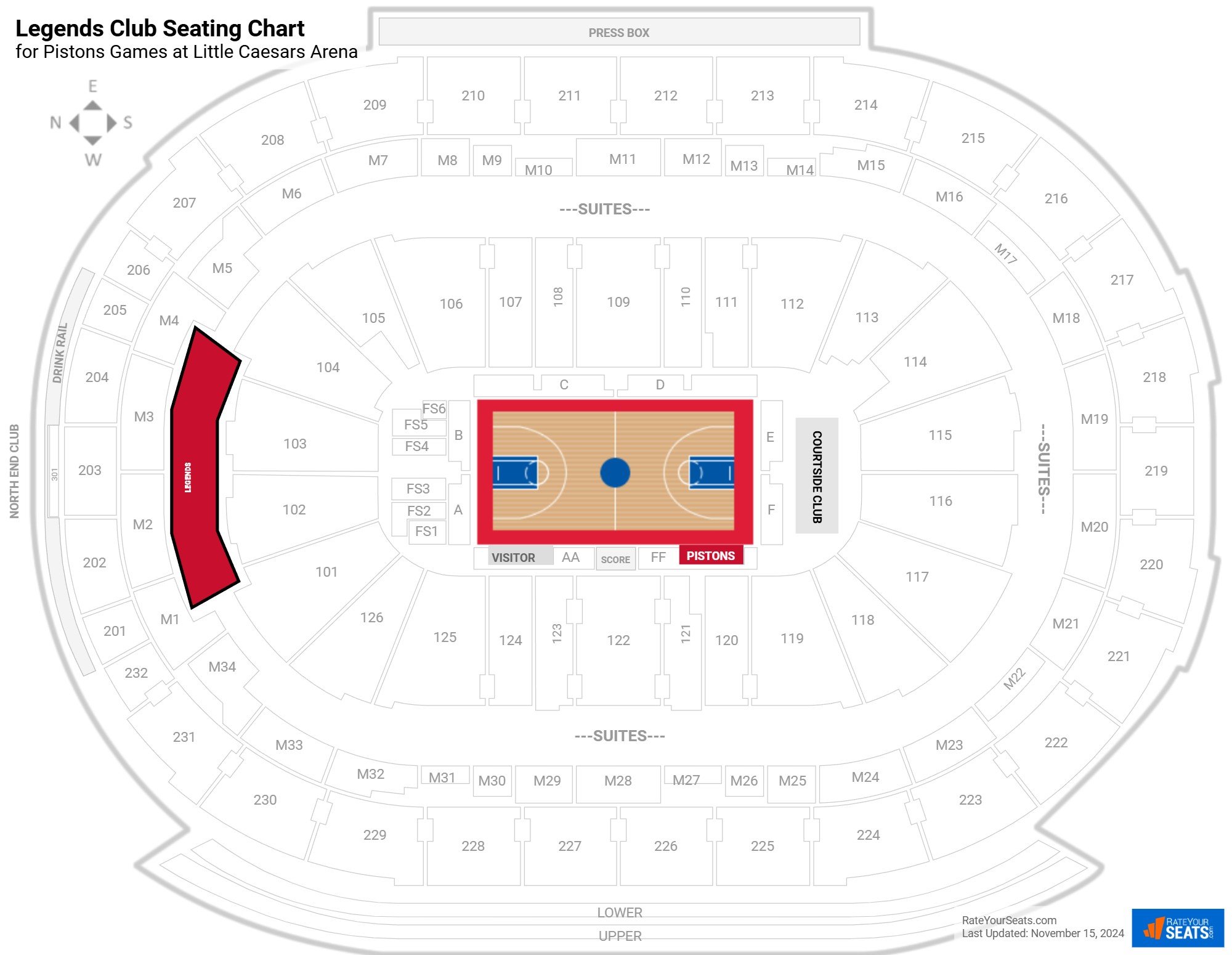This image features a detailed Legends Club Seating Chart for Pistons games at Little Caesars Arena. The orientation is provided by a compass beneath the title, with North to the left, East upward, South to the right, and West downward.

At the top, the blue-shaded press box is prominently marked, and the North End Club is noted at the far left. The chart outlines various seating sections, prominently displaying a central basketball court. Key features include the center circle and designated basket zones, clearly indicated with circles. Visitor and Pistons sections, along with scoring details, are also highlighted.

The seating layout begins with sections closest to the court, labeled A, B, C, D, E, F, AA, and FF, aligning with cutouts for the Pistons and visitors. The 100 ring of seats starts from section 101 at the bottom left, looping through to section 116 at the South side, behind one of the baskets. Notably, section 109 is at the top center, directly aligned with the center court, while sections 115 and 116 provide premium views from the South end.

Descending from there, the 122 section marks the center court area on the North side, flanked by suites and the M-sections. The middle tiers include M1 through M28, with M11 and M28 offering prime center court views, and M19 and M20 situated behind the baskets.

Further out, the 200 ring encircles the arena, providing additional seating options and a comprehensive view of the action below. A red area suggests an exclusive VIP section, strategically placed for optimal game viewing. This seating chart meticulously details the layout of seats, ensuring fans can locate their preferred spots for a stellar game experience.